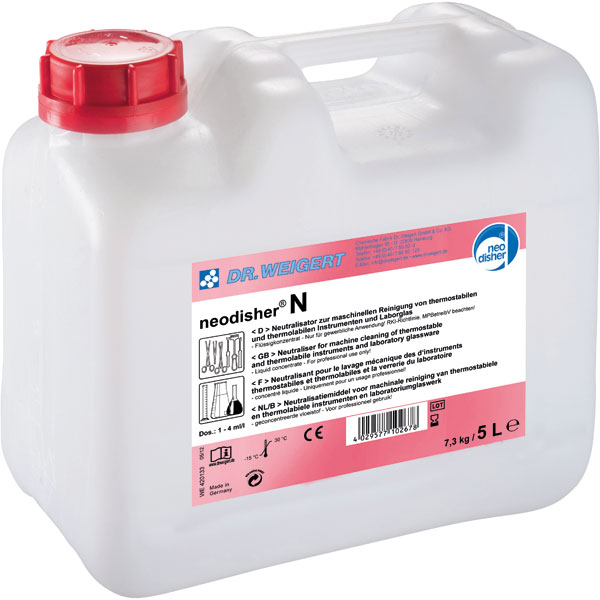The image showcases a close-up of a clear plastic 5-liter jug containing a transparent liquid, set against a solid white background. The jug, shaped like a rectangular prism, has a red twist cap on the upper left side and a horizontal handle on the upper right side. The jug is slightly angled to the left in the photograph. 

The front of the container features a prominent label divided into three sections: pink bands at the top and bottom, and a white section in the middle. In the upper left corner of the label, "DR. WEIGERT" is written in bold blue capital letters, accompanied by a small blue and white logo. In the upper right corner, there is a blue and white circular symbol with "Neodisher" inscribed in blue letters on a white background. Below this, the central white section displays "Neodisher" in black text with a large capital 'N'. 

The label also includes multiple small text blocks and symbols, some featuring illustrations of tools and lab equipment like flasks and beakers, indicating various certifications and product details in different languages. The bottom pink section contains a barcode in the center and the weight and volume specifications, "7.3 kg, 5 liter, E," in the lower right corner.

Overall, the image provides a detailed view of the jug and its labeling, emphasizing the branding and product information clearly.